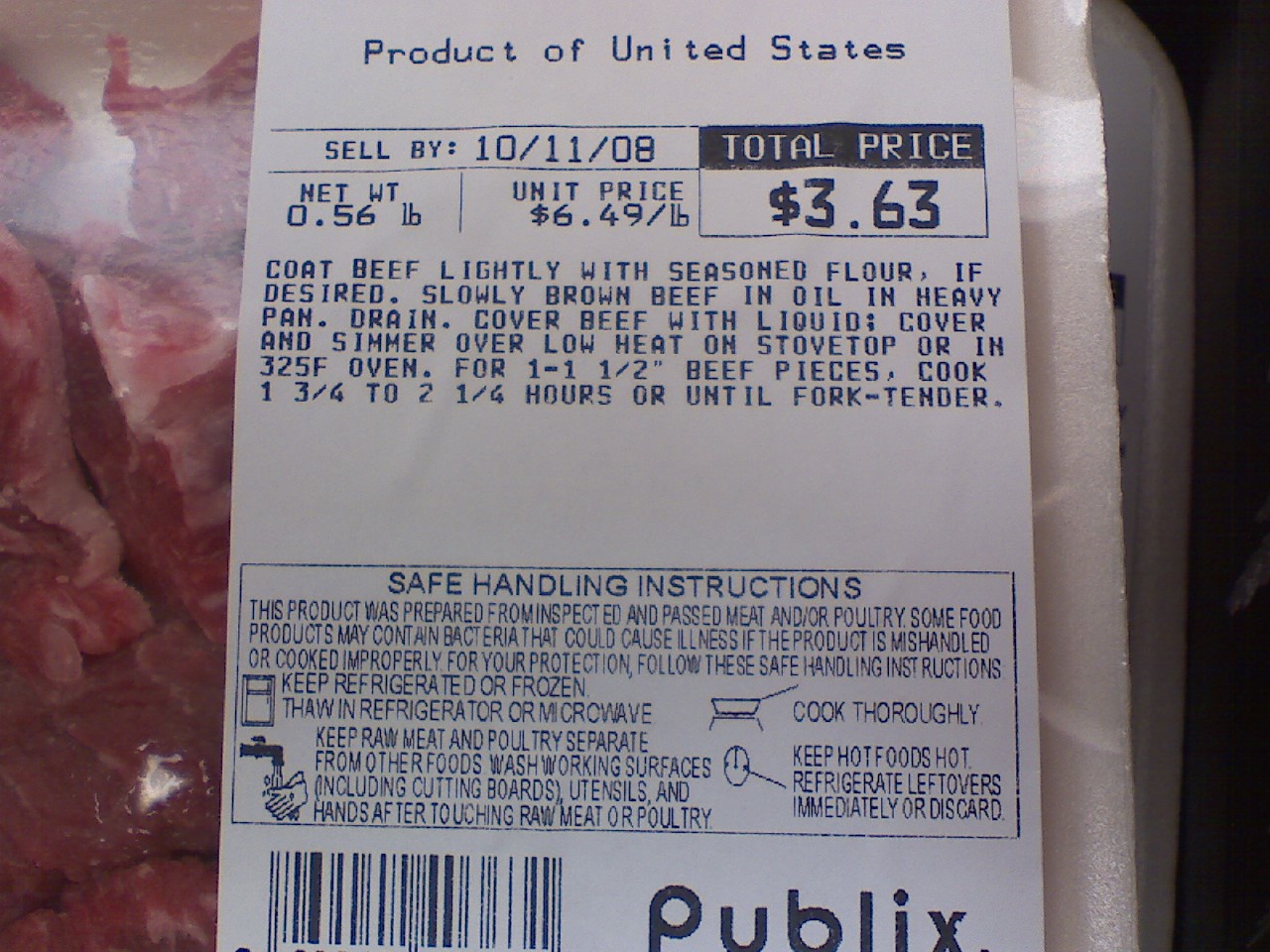This detailed image depicts a close-up photograph of a packaged meat product from Publix grocery store. The meat appears to be cut beef pieces, red in color with small amounts of white fat, encased in a clear plastic wrap atop a white styrofoam tray. The label occupies a significant portion of the image and is printed in black text on a white background.

The upper section of the label reads "Product of United States" and "Sell by 10-11-08." It also specifies the pricing details: a total price of $3.63, with a unit price of $6.49 per pound, and a net weight of 0.56 pounds. 

Below these details, the label provides cooking instructions. It advises to coat the beef lightly with seasoned flour, slowly brown it in oil in a heavy pan if desired, drain, cover the beef with liquid, and simmer over low heat on the stovetop or in a 325°F oven for 1 to 1.5 hours. For beef pieces, the cooking time extends to 1.75 to 2.25 hours, or until fork-tender.

Additionally, the label includes safe handling instructions, emphasizing the necessity of cooking the raw meat thoroughly, keeping hot foods hot, refrigerating leftovers immediately or discarding them, and maintaining separate work surfaces for raw meat and other foods to avoid cross-contamination. It also advises washing hands, cutting boards, and utensils after contact with raw meat.

In the lower right corner of the label, a partial view of the store name "Publix" is visible, confirming the retailer, although the bottom portion of the name is cut off. The lower left corner contains a black and white UPC barcode, though the numerical code itself is not visible.